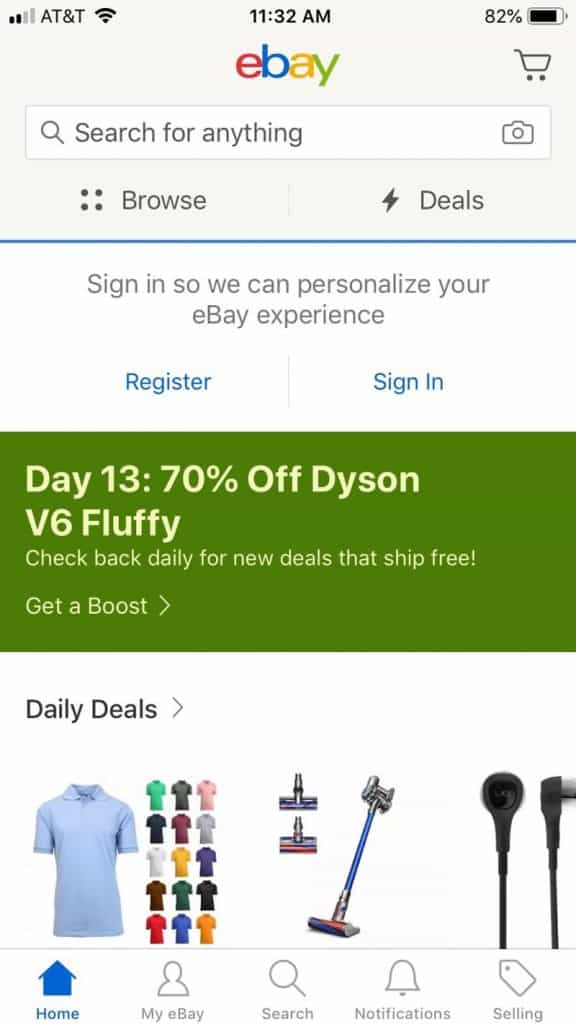A detailed screenshot of the eBay app displayed on an iPhone. The status bar at the top shows indicators for signal strength (bars), carrier (AT&T), Wi-Fi connection, the current time (11:32 am), and battery life (82%). Below this, the eBay logo is prominently featured, accompanied by a shopping cart icon on the right-hand side. 

Just beneath the header, the phrase "Search for anything" appears above a search bar, which includes a camera icon for image-based searches. Directly beneath, options to "Browse" or "Browse deals" are visible, separated by a thin blue line.

Further down, a prompt invites users to "Sign in so we can personalize your eBay experience," with buttons to either "Register" or "Sign in." 

Prominently featured in a green rectangular banner is an advertisement stating, "Day 13, 17% off Dyson V7 Fluffy. Check back daily for new deals that ship free," alongside a clickable button labeled "Get a boost."

Below the advertisement, a section titled "Daily Deals" showcases images of various items: a collection of multi-colored polo t-shirts, a Dyson vacuum cleaner, and a pair of wired headphones. 

At the very bottom of the screen, a navigation bar offers quick access to different sections of the app: "Home," "My eBay," "Search," "Notifications," and "Selling."